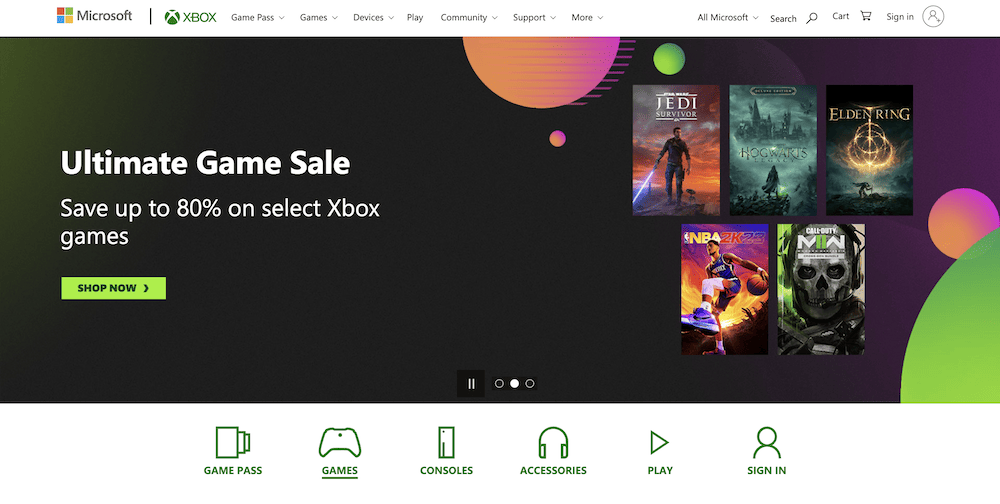This is a detailed screenshot of the Microsoft Game Store interface. In the top left corner, the iconic Microsoft logo, composed of four colorful squares (red, green, blue, and yellow) forming a larger square, is prominently displayed. To its right, the word "Microsoft" is written in a sleek black font. Adjacent to this, the Xbox logo is featured—a green circle with a white 'X' in the center—and beside it, "XBOX" is boldly written in green, all capital letters. 

The interface is organized with various categories extending from the left towards the right. On the far right, user's account information, including their cart and profile icon, is visible. Below this header area, a large rectangular background transitions from black on the left to a deep purple on the right, highlighting the store's sleek design.

Five featured games are displayed towards the right side against this background. These include titles themed around Star Wars, Hogwarts, "Elden Ring," and "NBA 2K." Another game features a menacing character with metallic skin, possibly named "IVAN," although the title is somewhat difficult to read due to its small font and tight lettering.

Below this section, a navigational menu is present with dark green icons and text. Categories here include "Game Pass," "Games" (which is currently selected and underlined in green), "Consoles," "Accessories," "Play," and "Sign In." This polished and functional layout showcases various sections of the Microsoft Game Store, inviting users to explore its diverse gaming content.